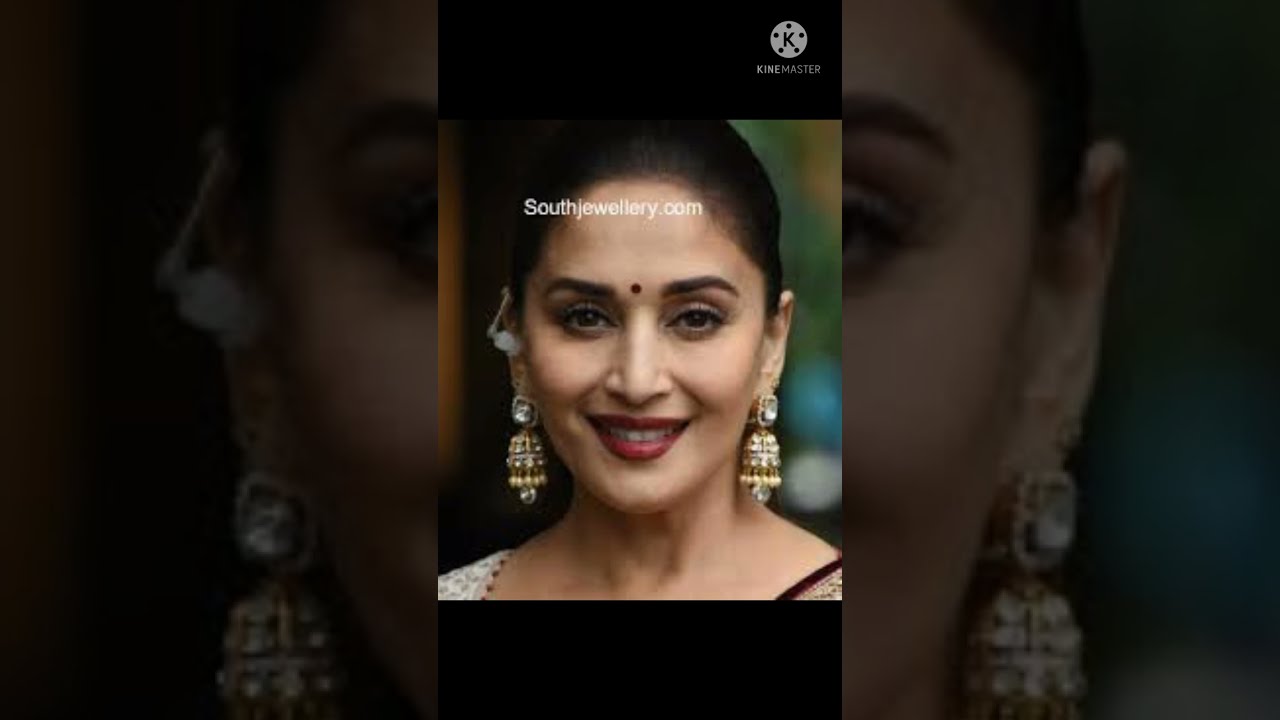The photograph features a South Asian woman, likely of Indian descent, captured in a headshot style with a black border at the top and bottom. Her face is centered in the frame, characterized by light brown skin, dark brown to black hair pulled tightly back, and a traditional red bindi on her forehead. She has deep red lipstick on and is smiling warmly at the viewer. Her striking earrings are long, dangling, and made of gold and possibly diamonds or crystals, forming a bell-like shape. The woman is dressed in what appears to be a sari, with a glimpse of a white blouse visible on her right shoulder and some black and gold fabric on her left. Superimposed at the top of her forehead in white text is the URL "southjewelry.com," and in the upper right-hand corner is a white circle with a "K" logo, accompanied by the text "Kinemaster." The background features a muted, enlarged, and zoomed-in image of the same woman, adding depth to the composition.